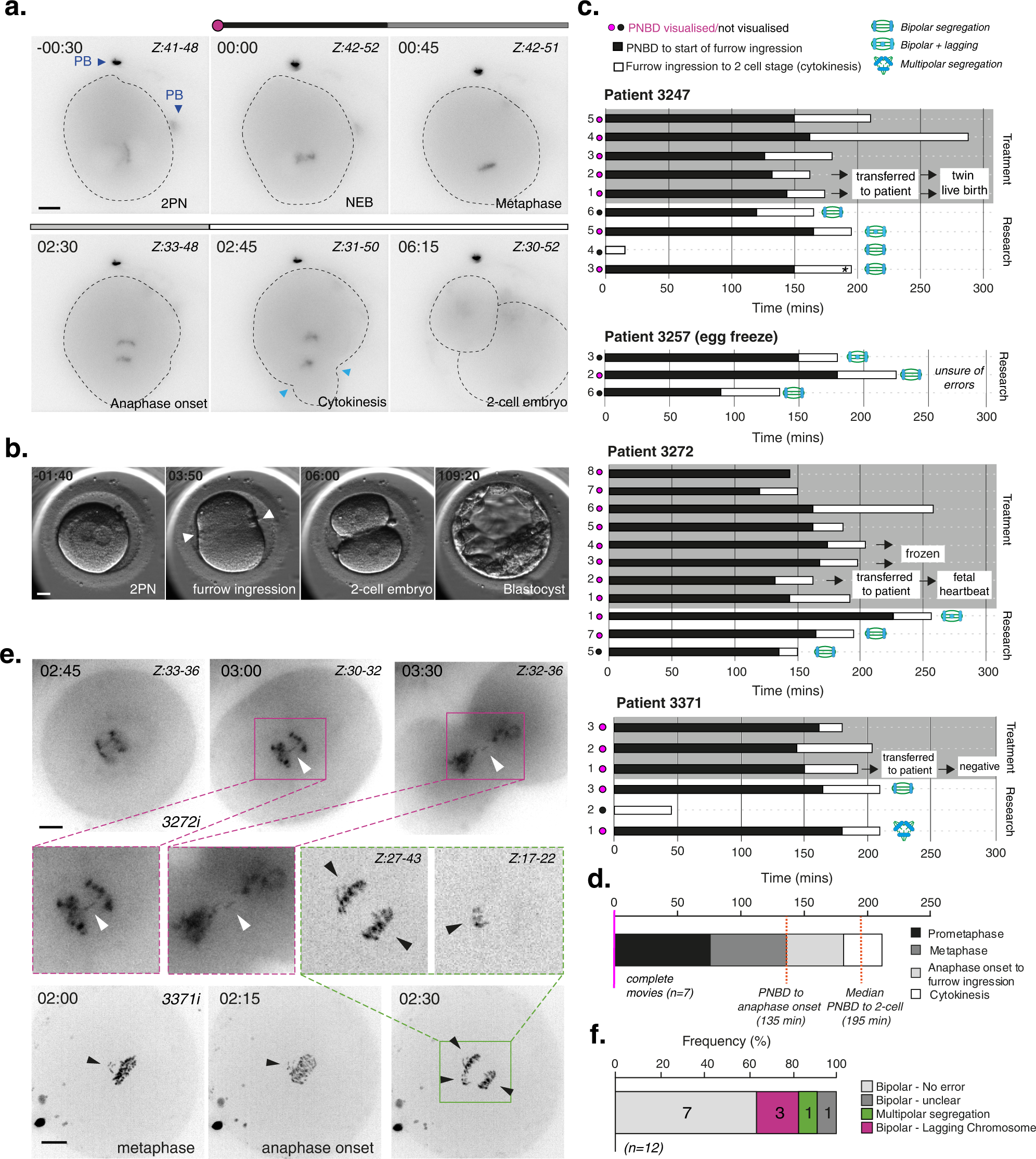The photograph displays a detailed medical diagram, likely related to embryonic development, containing various microscopic images and patient data. The diagram is segmented into labeled boxes, A through F, each depicting different stages and information regarding patient embryos. Box A includes images of embryos at early stages, such as metaphase and anaphase onset, and a two-cell embryo. Box B presents similar images, featuring embryos in a darker, more liquid state. Sections C, D, and F contain patient numbers, including 3272, 3371, and 3257, with corresponding line graphs and charts illustrating details about birth, embryo transfer, and egg freeze status. Lastly, Box E displays additional microscopic photos of embryos, showcasing stages like metaphase and anaphase onset, contributing to a comprehensive visual display of the embryos' development over time.